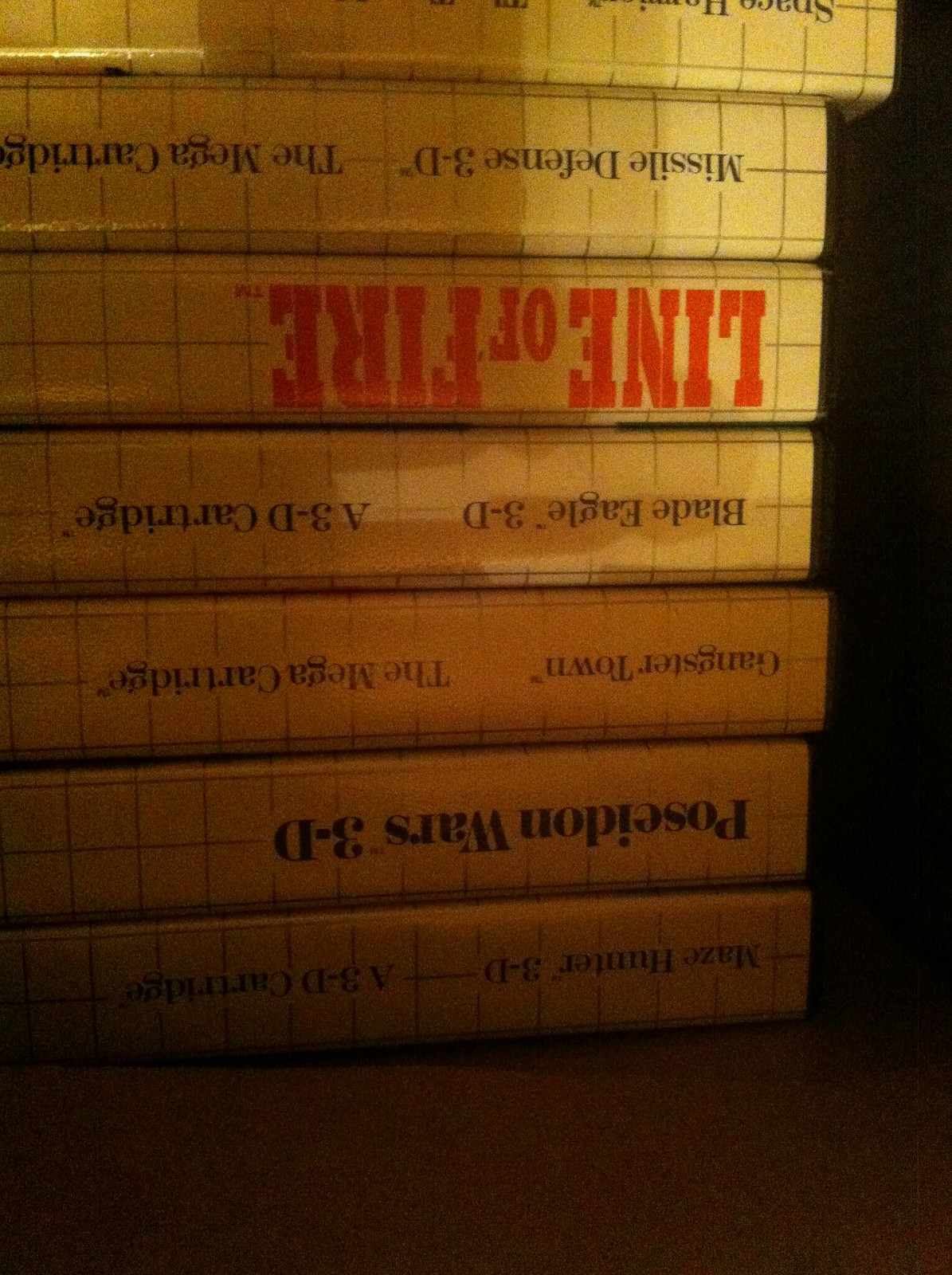In the photograph, a dark room creates an almost black void-like backdrop, making the back wall invisible. A dark brown table surface dominates the foreground, its material indistinguishable due to the low light. On this table sits a stack of six cases, initially described as books. Each case is light brown with a dark square grid pattern on the spines. Titles on these spines, written in a mix of black and red fonts, are clearly visible upside down. The titles read: Maze Hunter 3D, Poseidon Wars 3D, Gangster Town, Blade Eagle 3D, Line of Fire (in red letters), and Missile Defense 3D. Given the repeated mention of "The Mega Cartridge" and "3D Cartridge," these "books" are revealed to be retro video game cases for an early 3D gaming system. The distinct titles and patterns suggest a nostalgic collection ready for exploration.